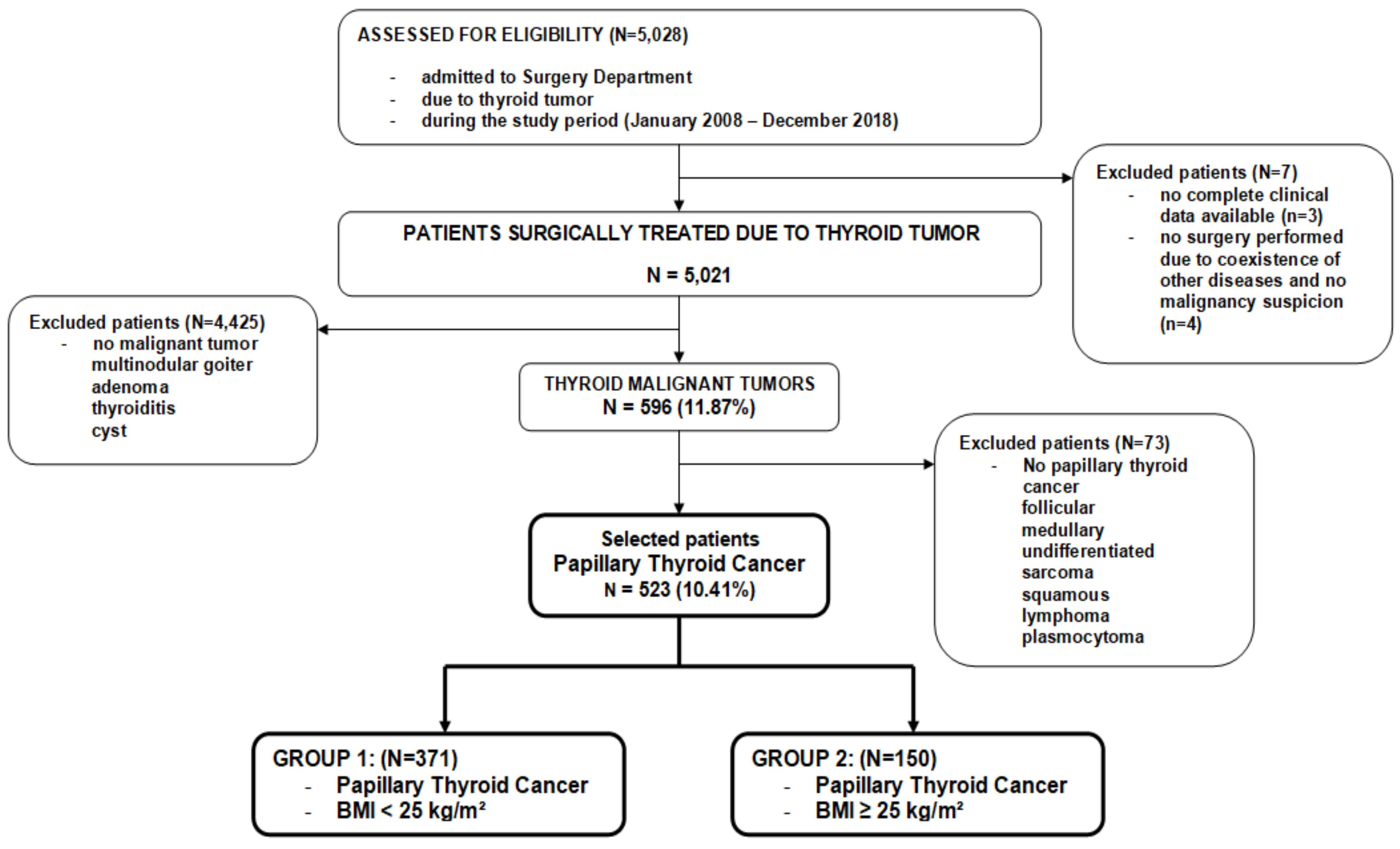The flowchart provides a detailed step-by-step overview of the diagnosis and treatment pathway for patients presenting with thyroid tumors, tracked over the study period from January 2008 to December 2018. At the top, the chart starts with assessing 5,028 patients for eligibility, specifying that they were admitted to the surgery department due to suspected thyroid tumors. These patients are then categorized: 5,021 patients were surgically treated for thyroid tumors, while 7 were excluded due to incomplete clinical data (3 patients) or non-surgical cases resulting from coexistence of other diseases and no malignancy suspicion (4 patients).

From the surgically treated group, another categorization occurs: 4,425 patients were further excluded because they did not have malignant tumors, displaying conditions such as multinodular goiter, adenoma, thyroiditis, or cysts. This left 596 patients with confirmed malignant thyroid tumors, making up 11.87% of the original cohort. Among these, additional exclusions (73 patients) were made for those showing non-papillary types of thyroid cancer, such as follicular, medullary, undifferentiated sarcoma, squamous, lymphoma, or plasmocytoma. 

Finally, 523 patients were identified with papillary thyroid cancer, representing 10.41% of the initial group. These patients were then divided into two groups based on body mass index (BMI): Group 1 consisted of 371 patients with a BMI of less than 25 kg/m² and Group 2 included 150 patients with a BMI greater than or equal to 25 kg/m².